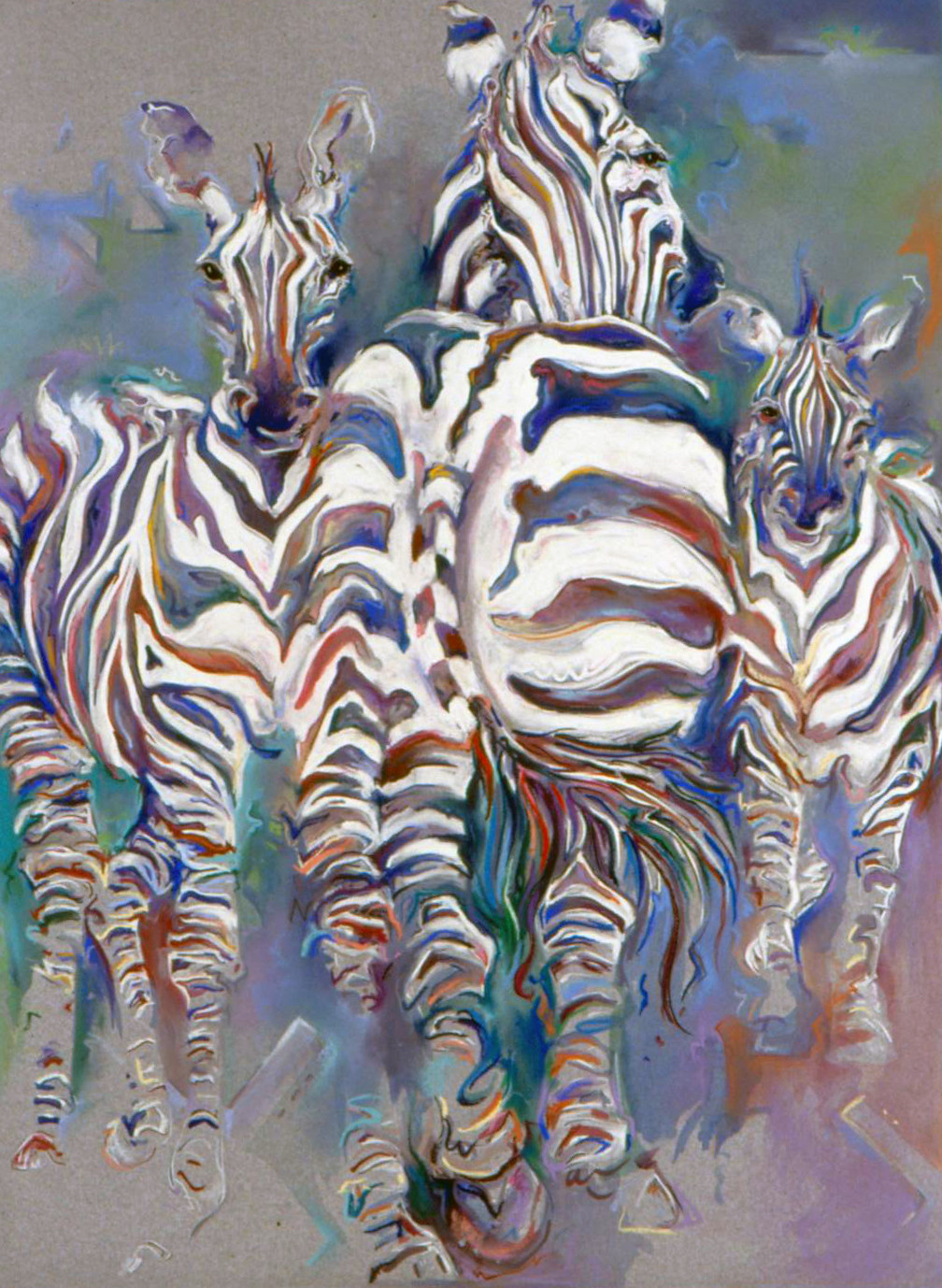The painting features a vibrant and colorful depiction of three zebras, each adorned with a mix of stripes in blue, green, purple, yellow, red, orange, and brown hues, creating a visually arresting, almost watercolor-like effect. The background transitions from a dark gray-blue at the top, blending with other colors to form an abstract style, to a lighter gray toward the bottom. The central zebra is positioned with its back to the viewer, revealing its rainbow-colored tail and rounded ears, while the zebras on either side face forward, their vivid stripes reflecting in the striking hues of the painting. The legs of the right-most zebra gradually fade into the background, adding to the artwork's surreal and dreamy atmosphere. The zebras dominate the composition, their proximity and overlapping figures lending a dynamic, almost crowded appearance to the scene.